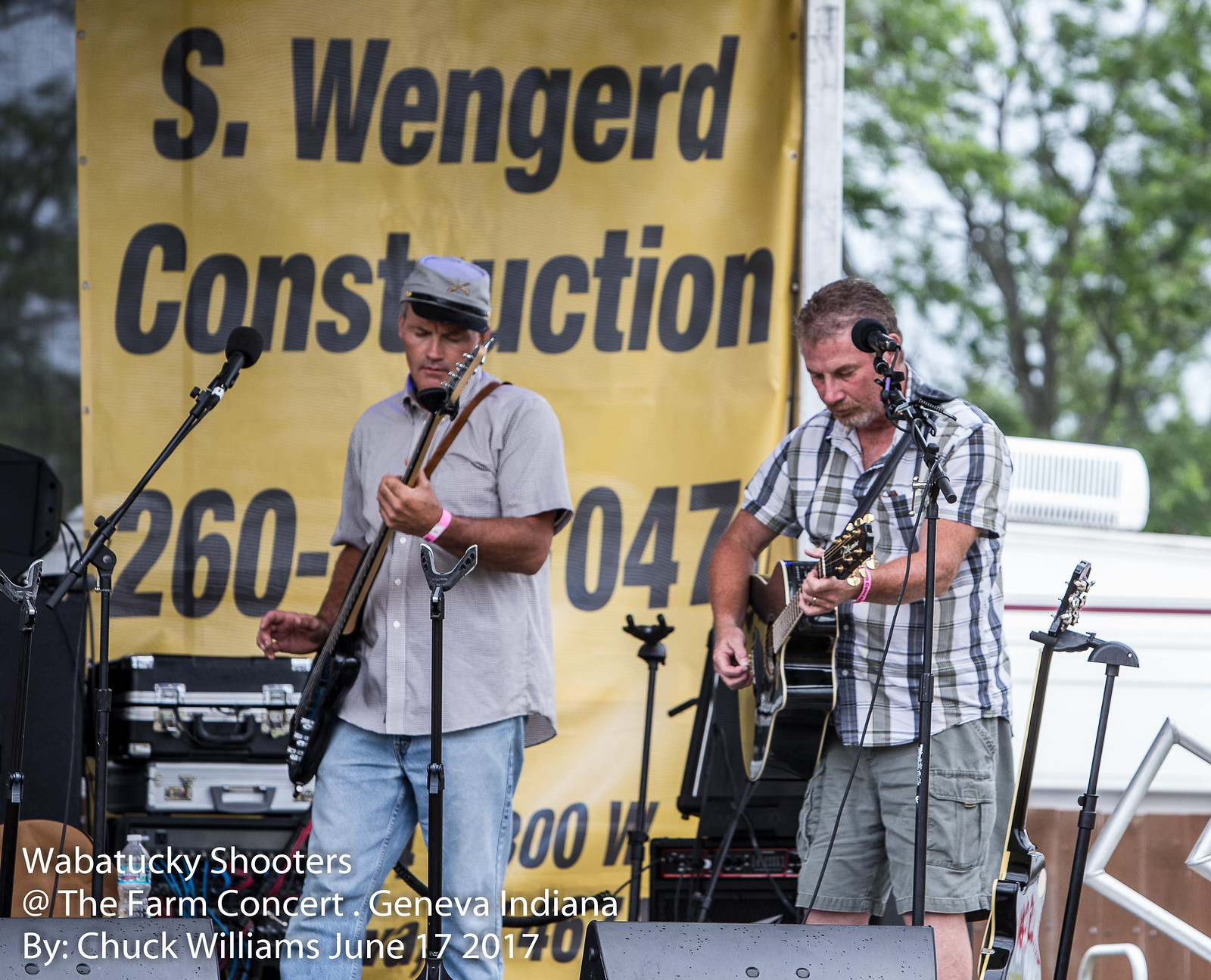In this vibrant outdoor photograph, captured at the Farm Concert in Geneva, Indiana, on June 17, 2017, by Chuck Williams, we see two middle-aged Caucasian men performing on a stage marked by a large yellow banner in the background. The banner reads "S. Wengerd Construction" in dark letters, and displays a partially visible phone number "260...047." The stage is set against a scenic backdrop of trees and sky, adding to the rural charm of the scene. 

The performer on the left, dressed in a tan shirt, denim jeans, and a gray Confederate cap, strums a black electric guitar while looking down at his instrument. Beside him, the musician on the right, clad in a plaid short-sleeve shirt and light-colored cargo shorts, plays an acoustic guitar, also focused on his strings. Both men stand before microphones, fully immersed in their performance. 

The stage is equipped with various musical gear, including subwoofers, amplifiers, and additional guitar stands—one empty in front of the man with the electric guitar and another to the right holding a guitar next to the plaid-shirted musician. The detailed caption at the bottom of the photograph reads, "Wabatuckee Shooters at the Farm Concert, Geneva, Indiana, by Chuck Williams, June 17, 2017," lending a personal touch to this snapshot of a simple yet captivating musical moment.